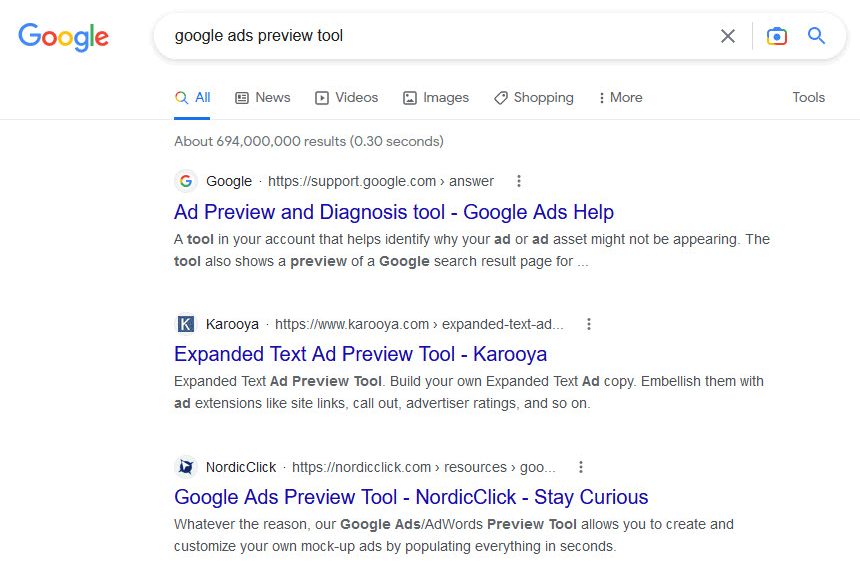A computer screen displays a Google search for "Google ads preview tool," revealing three distinct results. The first link is from Google Support, offering detailed guidance on the Ad Preview and Diagnostic Tool. It explains that the tool, available within Google Ads accounts, helps identify reasons why an ad or ad asset may not be appearing, and includes a preview of a Google search result page. The second result is from www.karua.com, advertising their Expanded Text Ad Preview Tool. This tool allows users to build and embellish their own expanded text ad copy with extensions such as site links, callouts, and advertiser ratings. Lastly, the third result is from nordicclick.com, promoting their Google Ads Preview Tool. The Nordic Click tool emphasizes the ability to create and customize mock-up ads quickly by populating all the necessary fields in seconds.